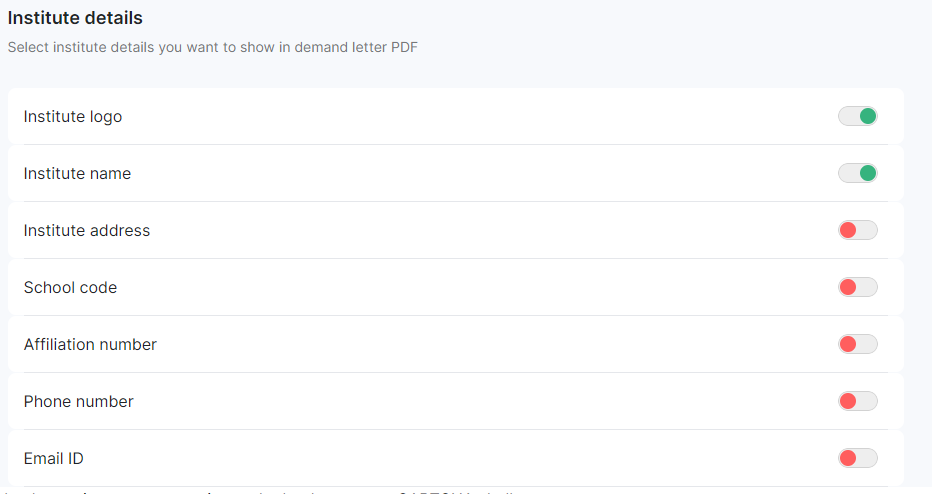**Category: Websites**

**Caption:** 

This webpage is dedicated to configuring settings for a Demand Letter PDF under the section "Institute Details." The top gray header prominently displays the title "Institute Details." Below, users can select which institute details to include in the PDF. The options listed include:

- Institute Logo (On - shown in green)
- Institute Name (On - shown in green)
- Institute Address (Off - shown in red)
- School Code (Off - shown in red)
- Affiliation Number (Off - shown in red)
- Phone Number (Off - shown in red)
- Email ID (Off - shown in red)

Each option is separated by a line, offering a clear distinction between sections. The interface is minimalist, utilizing a gray, white, and black color scheme, with status indicators in green and red. There are no additional elements, labels, or informational text on the page, leaving the purpose and context of the page, website, and type of demand letter unspecified.